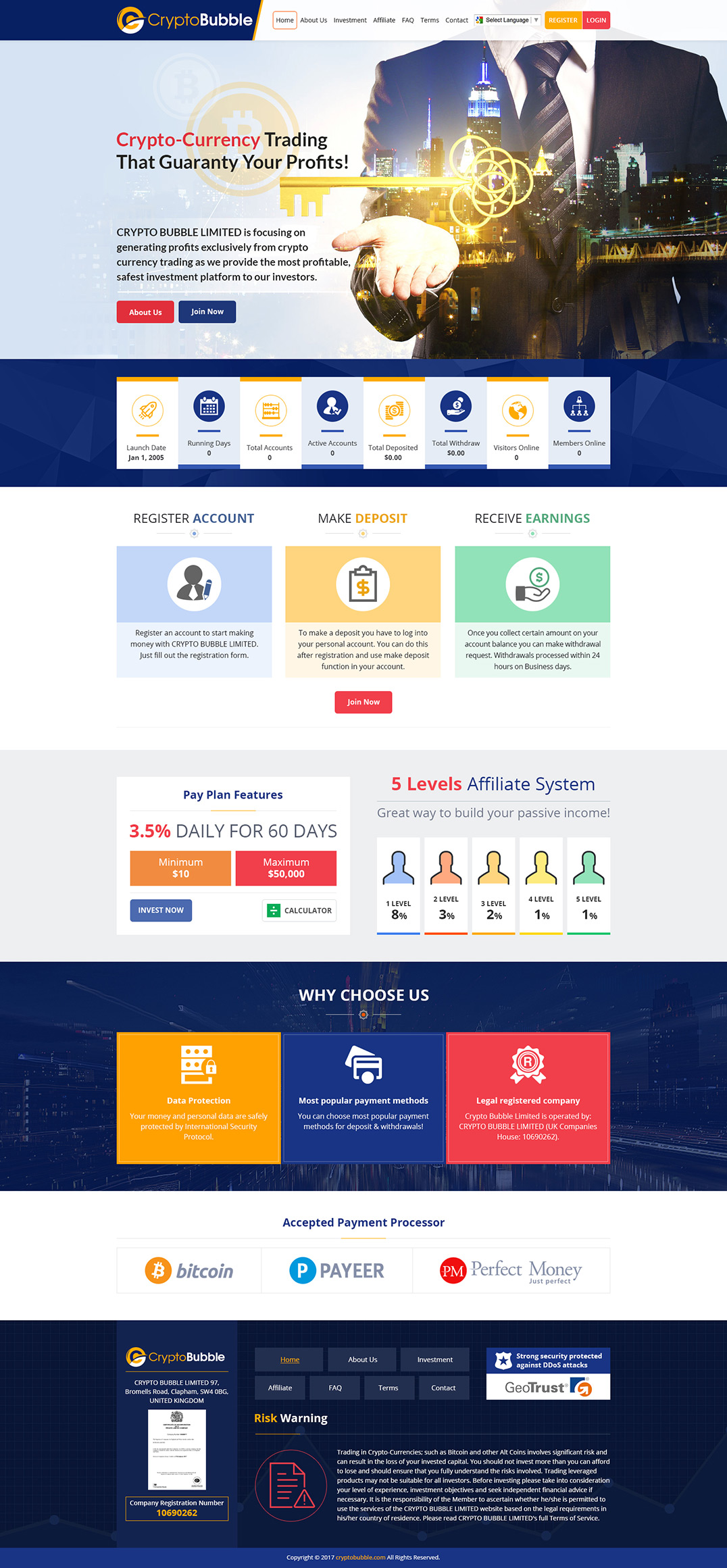This image is a detailed screenshot of a webpage layout. At the top of the page, a distinctive rectangular section prominently features a blue strip that transitions to white about halfway across. Centrally positioned within this section is a photograph showing the torso of a man in a business suit, with his right hand extended, palm up.

Beneath this, there is a large blue rectangle containing several vertical rectangles that alternate in color between white and blue. Each of these rectangles is adorned with an icon and small text. Following this blue section is another larger rectangle with a white background, housing three centered vertical rectangles. These rectangles are differentiated by their colors: blue on the left, yellow in the middle, and green on the right, each accompanied by a title, an icon in the center, and small black text below.

Further down the page, there is a red centered rectangle followed by a gray rectangle that houses two boxes. The left box contains an orange section on its left side and a red section on the right, with some text positioned above and a blue rectangle in the lower-left corner. The right box displays a title at the top, a line of black text, and five vertical rectangles below, each featuring an abstract icon resembling a person. 

Below this section is another blue rectangle that contains four smaller squares: an orange square on the left, followed by a blue square, a red square in the middle, and another blue square with extensive text. Along the left side of this layout is a vertically oriented rectangle with a centered white square.